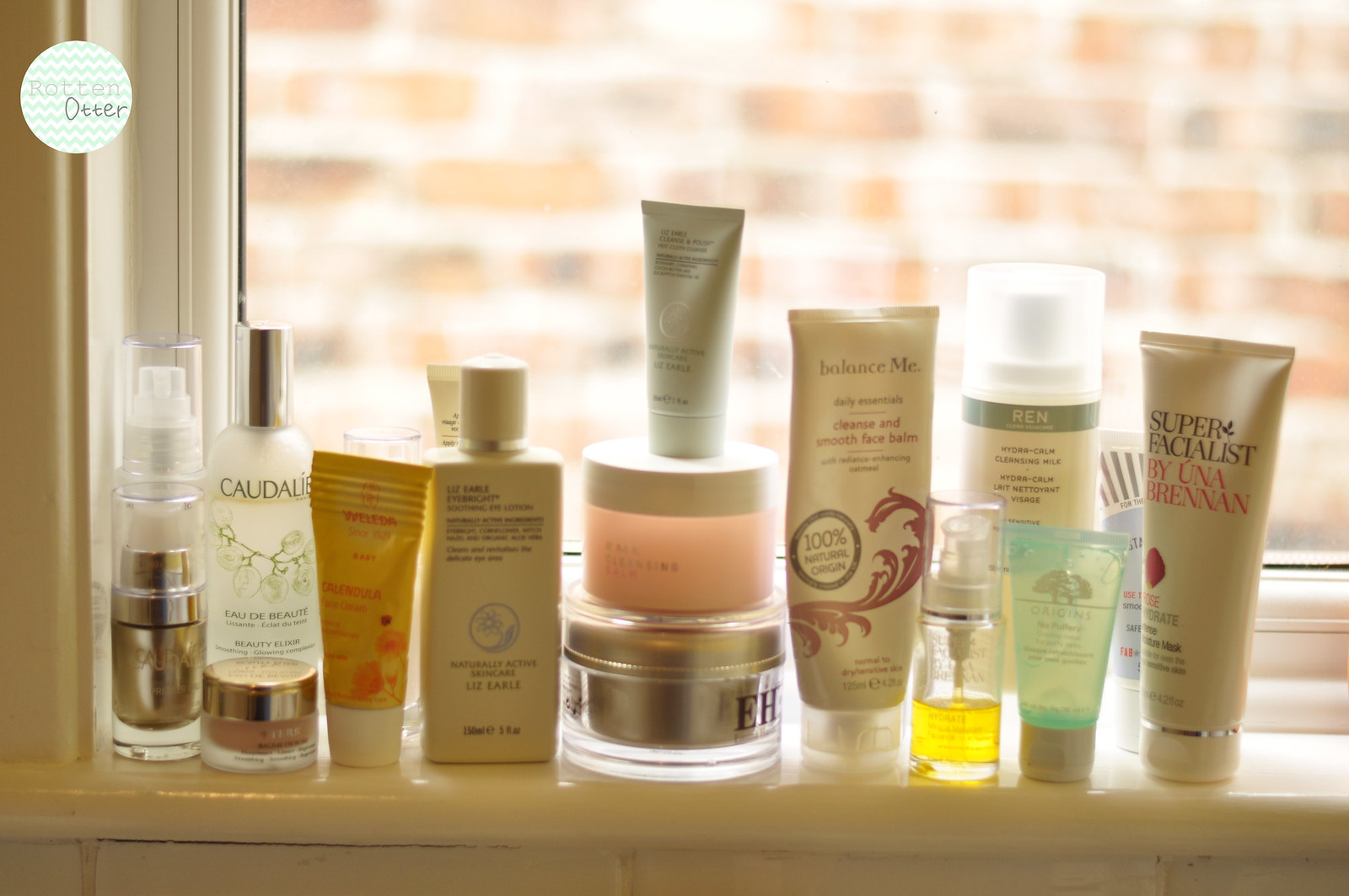In the image, several beauty products are arranged on a bathroom windowsill with a closed window in the background. The background is blurred, revealing a red brick wall outside. The promotional label "Super Facialist" is prominently displayed on one of the products. Among the items, there is a partially used product with a light orange or yellowish hue, adding a touch of color to the scene. The arrangement includes a silver circular container, a clear container with shades of pink and off-pink, and a small tube perched on top. Additionally, a potential perfume or other facial product is visible. The windowsill sits above a tiled surface, reinforcing the bathroom setting. Lastly, a container labeled "Balance Me" can also be seen among the assortment of beauty products.